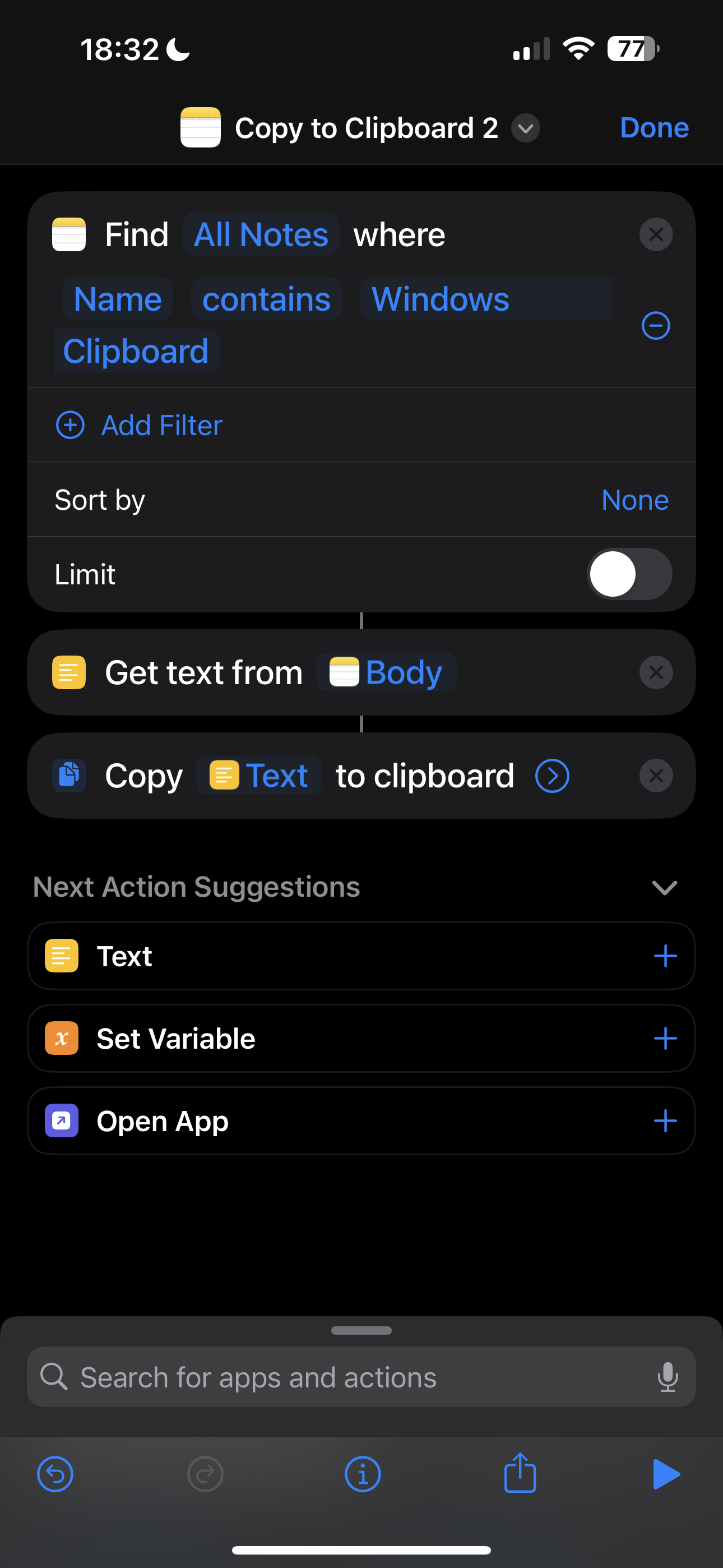This image showcases a screenshot of a mobile application with a predominantly dark theme. The screen features a black background complemented by a dark grey header and footer. 

The dark grey header prominently displays a centered title, "Copy to Clipboard 2," in white text. Accompanying the title is a medium grey circle containing a light grey downward-pointing arrow. On the left side of the title, there is a notebook emoji, while the right side displays blue text that reads "Done."

Below the header, the black background hosts several medium grey rectangles with rounded corners, forming a structured layout. The largest rectangle at the top includes a header line with the text "Find" in white, "All Notes" in blue, and "Where" in white. This line is flanked by a duplicate notebook emoji on the top left and a medium grey circle with a dark grey 'X' on the top right.

The subsequent line features terms in blue text: "Name," "Contains," "Windows," and "Clipboard," followed by a blue donut icon with a blue minus sign on the right.

Separated by a thin medium grey line, the next line presents the blue text "Add Filter," accompanied by a blue donut with a blue plus sign on the left. Another thin grey line divides this from the subsequent row, which in white text says "Sort By," with "None" in blue text on the right.

The final entry in this section reads "Limit" in white text, boasting a selection button on the right. This button is depicted as a white circle on the left side of a medium grey pill-shaped slider extending to the right.

Overall, the image intricately details the UI elements and layout of the "Copy to Clipboard 2" application on a mobile phone, emphasizing its dark-themed design and structured functionality.